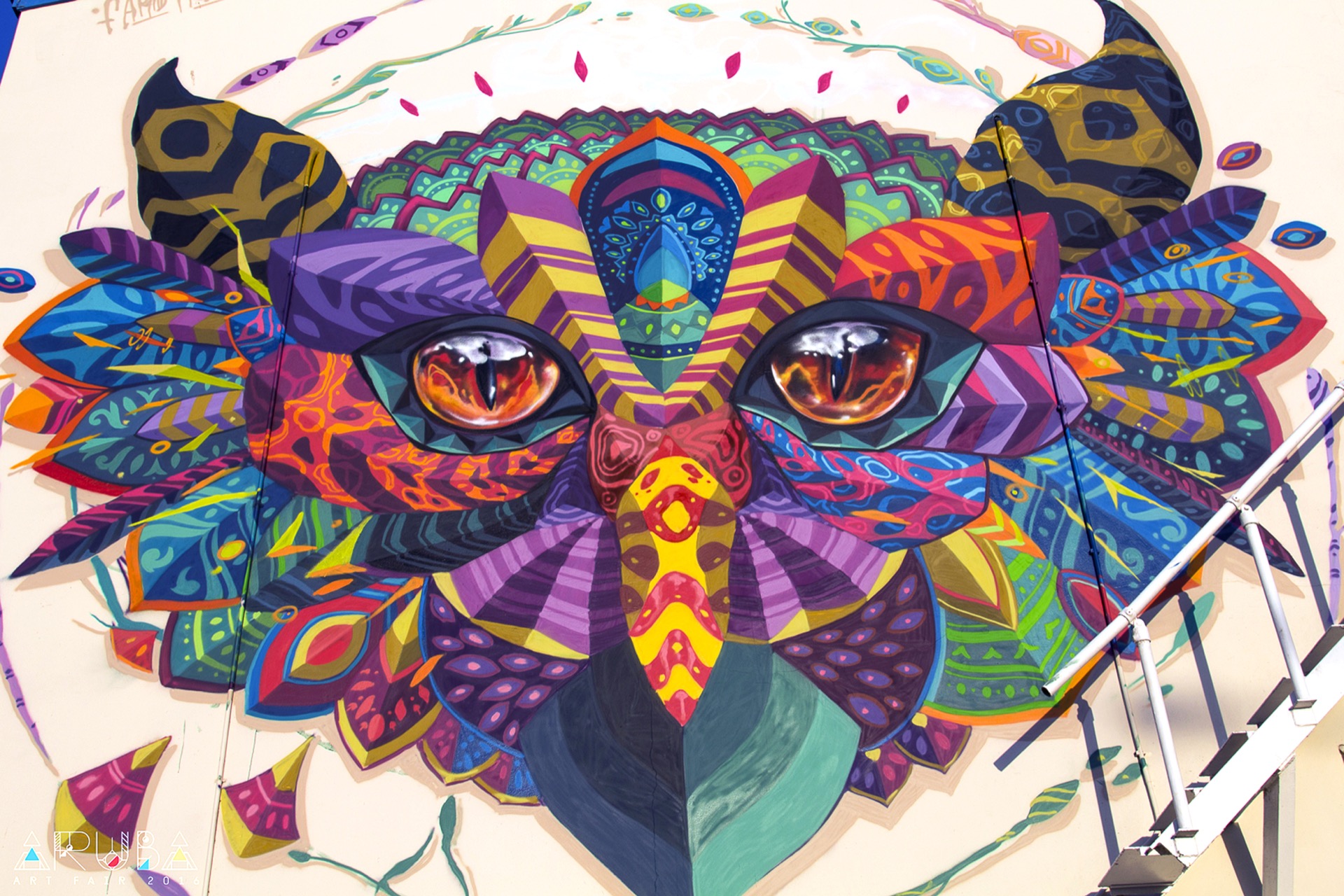This photograph captures a stunning mural adorning the side of a building, demonstrating an exquisite blend of artistic skill and possibly digital or AI-generated enhancements. The mural features an incredibly lifelike rendering of a bird's face, creating a striking focal point set against the cream-colored background of the wall. The artist has meticulously detailed the eyes and beak, imbuing them with a sense of realism and depth. Surrounding the central bird's face are intricately painted feathers, each uniquely colored and patterned, contributing to a vibrant and dynamic visual spectacle. Adding an element of urban contrast, a white metal staircase, resembling a fire escape, ascends alongside the mural, integrating a functional piece of architecture into the overall aesthetic of the artwork.